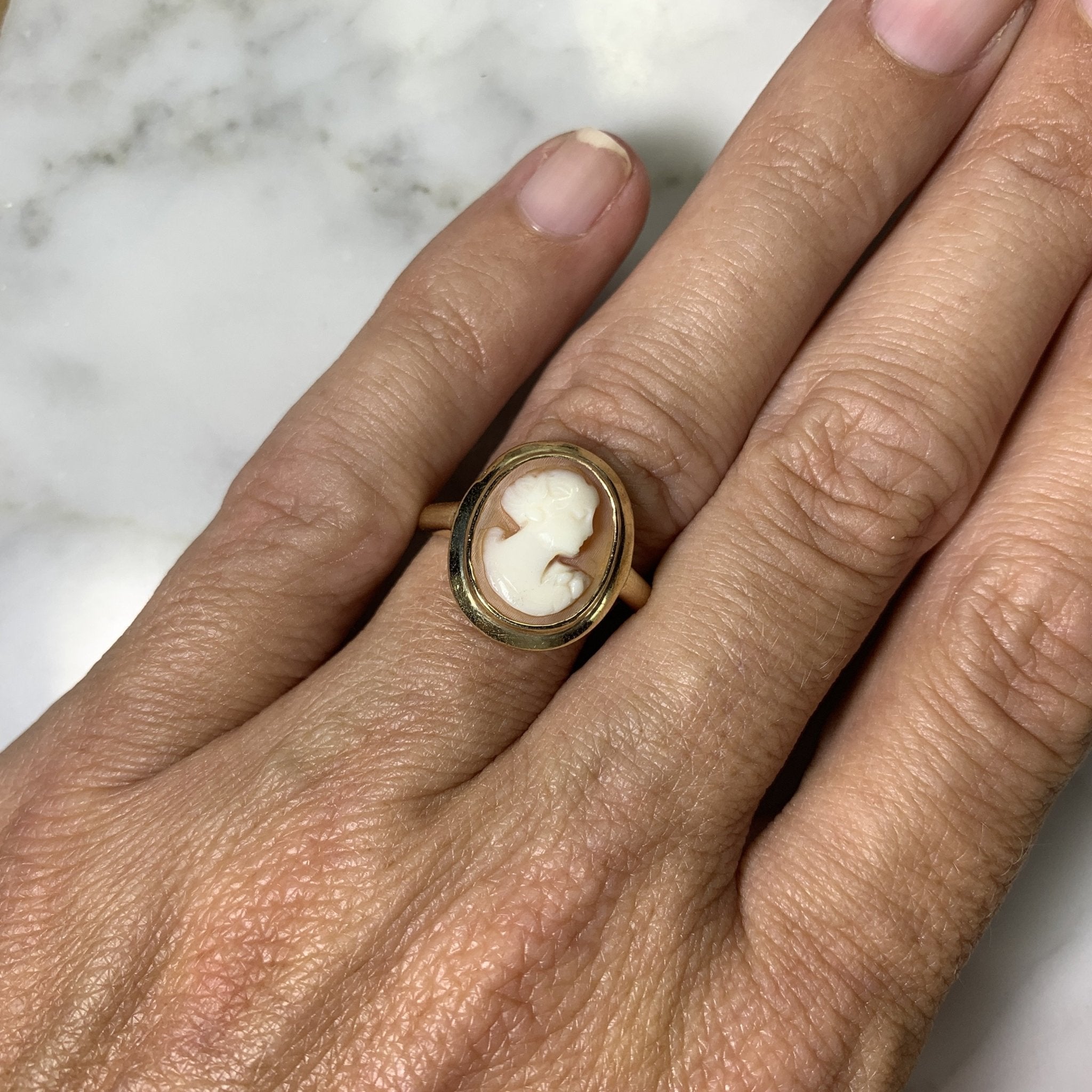The photograph is a close-up shot of a wrinkled, textured hand resting on a slab of marble, where only four fingers—the pinky and three partial fingers—are visible, while the thumb is not. The nails are generally well-manicured, except for the pinky nail, which appears a little unkempt and in need of a trim. The focus of the image is on a vintage-style, gold cameo ring worn on the ring finger. The ring is oval-shaped and features an intricately carved woman's head and shoulders made of white porcelain or marble. The woman, who has short, curly hair and a prominent chin, appears to have her eyes closed and is facing to the right. She wears what seems to be a vintage, frilly-style dress, lending an elegant and timeless charm to the ring.